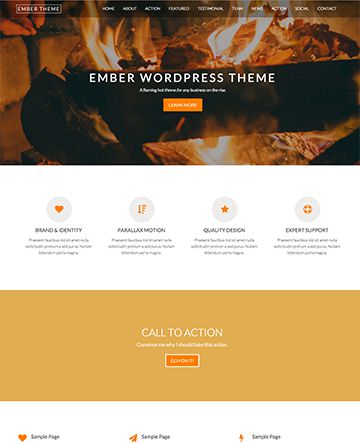The image is a web advertisement for the Ember WordPress theme. At the top of the screen, there is a brown color scheme featuring a photograph of a burning log. Superimposed in white text is "Ember WordPress Theme," under which there is an orange box that says "Learn More." Above this, in white text, are menu items from left to right: home, about, action, featured, testimony/testimonial, team, news, action, social, and contact.

The middle section of the webpage features a white area with four circles, each containing different icons: the first circle has an orange heart labeled "Brand and Identity," the second has an arrow pointing down with lines next to it labeled "Parallax Motion," the third circle has an orange star labeled "Quality Design," and the fourth features an orange and white globe labeled "Expert Support."

At the bottom of the page, there is a large gold rectangular area with white text that says "Call to Action," and below this, an orange clickable box, too blurry to read clearly but possibly saying "Go for it," "Learn More," "Next," or something similar. The primary colors used in the advertisement are white, black, tan, and shades of orange.